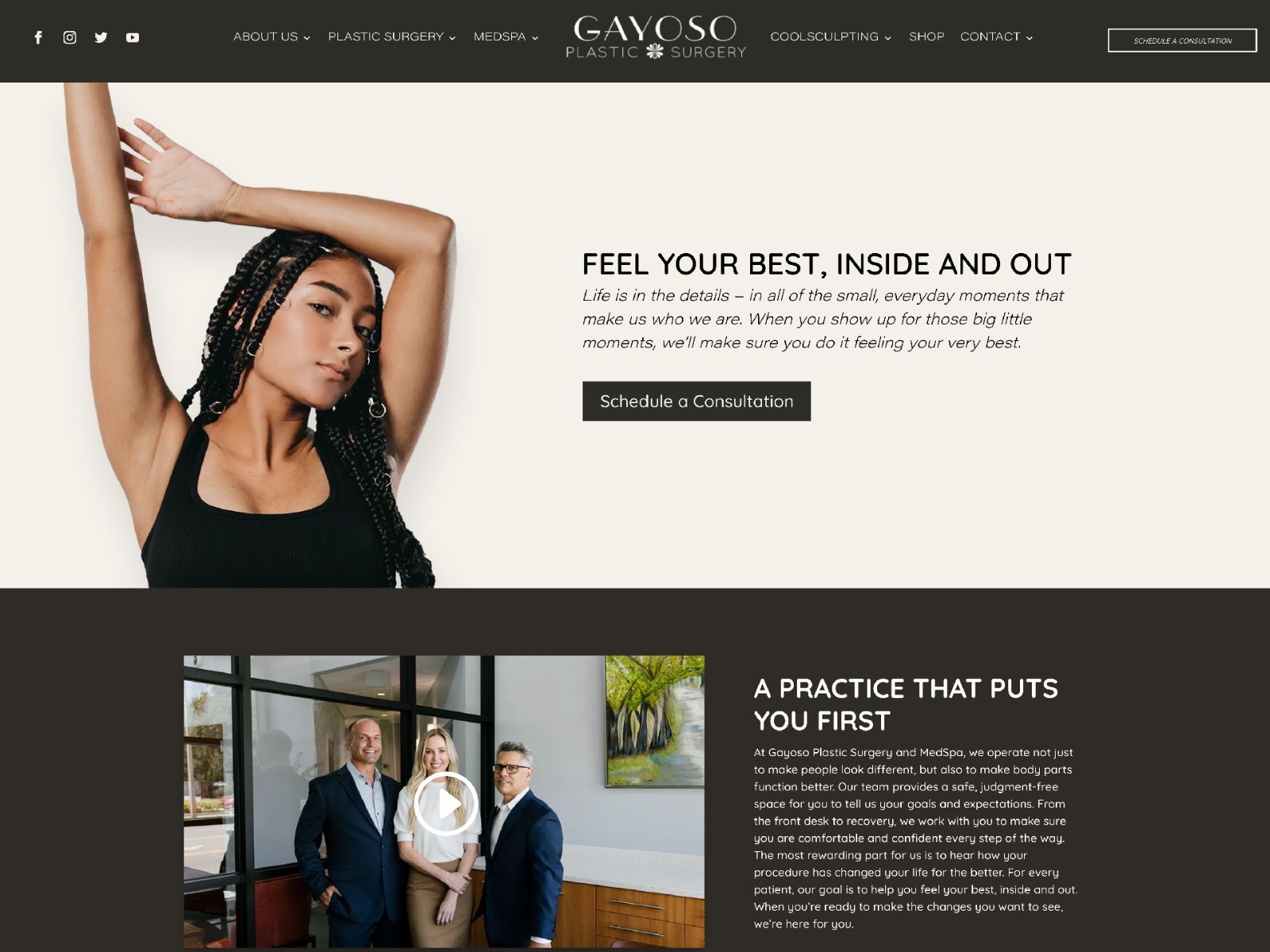**Detailed Caption for Govoso Plastic Surgery Website Image:**

This online rectangular landscape image, resembling the shape of most laptop screens, is an intricate depiction of the Govoso Plastic Surgery website layout. The image is sectioned into three horizontal rectangular areas:

**1. Header Section (Top 10%):**
- Background: Very dark brown or black.
- Upper Left Corner: Features standard social media icons - Facebook, an unidentified second icon, and Twitter.
- Center: The stylized text "GAYOSO" in all caps, with "PLASTIC SURGERY" beneath it in smaller letters. Between the words "PLASTIC" and "SURGERY" is an indistinct logo resembling an '8' with leaf-like shapes extending from the top and bottom.
- Pull-Down Menus: Positioned around the center, three on each side - 'ABOUT US,' 'PLASTIC SURGERY,' 'MED SPA' to the left, and 'COOL SCULPTING,' 'SHOP,' 'CONTACT' to the right. All except 'SHOP' have a downward-facing arrow.

**2. Main Section (Middle 50-60%):**
- Background: Light grayish-tan.
- Left Side: Image of an African American woman, visible from just below her breasts to above her head, wearing a sleeveless, very dark top. Her right arm is raised high, almost straight up, with her left arm bent at the elbow, resting across the top of her head. Her head tilts slightly to her left, but she maintains eye contact with the viewer. Her dreadlocks cascade down her right shoulder and in front of her left shoulder.
- Right Side: Bold all-caps text in dark brown-black font, stating "FEEL YOUR BEST, INSIDE AND OUT." Below this are three lines of italicized text. Further down, a clickable field in white font reads "SCHEDULE A CONSULTATION."

**3. Bottom Section (Lower 40%):**
- Background: Dark brown.
- Left Side: A video thumbnail displaying three people in an office setting, identifiable by a white play button in the center. The individuals include two men in dark blue suits without ties on the left and right, and a woman in the middle wearing a light top and brown skirt. The man on the right also wears glasses, and all three are looking at the camera.
- Right Side: Large bold white text in all caps reads "A PRACTICE THAT PUTS YOU FIRST." Beneath this, approximately 13 lines of smaller white text describe the practice, starting with "At Gayoso Plastic Surgery and Med Spa...", providing detailed information about the services and philosophy of the practice.

This detailed layout highlights the structured, professional, and appealing design of Govoso Plastic Surgery's website, emphasizing both visual aesthetics and informational clarity.